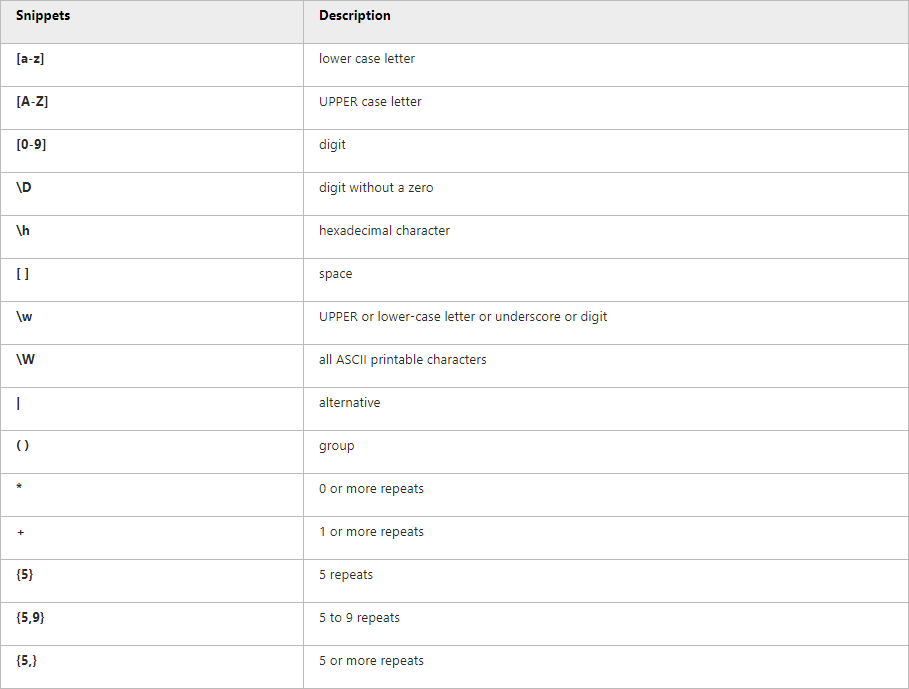The image features a table formatted like an Excel spreadsheet, comprising two columns where the right column is double the width of the left. The table consists of evenly spaced rows, all white except for the top row, which is gray. In the gray top row, the text is bold. In the left column, the text is also bold, unlike the regular text in the right column.

**Left Column:**
- Snippets (title)
- [a-d]
- [A-Z]
- [0-9]
- \D
- \h
- [\w]
- [\W]
- \l
- \L
- \(
- \.
- \+
- (5)
- (5,9)
- (5,)

**Right Column:**
- Lowercase letter
- Uppercase letter
- Any uppercase letter
- Digit
- Digit without zero
- Hexadecimal character
- Space
- Upper or lowercase letter or underscore or digit
- All ASCII printable characters (ASCII)
- Alternate group
- 0 or more repeats
- 1 or more repeats
- 5 repeats
- 5 to 9 repeats
- 5 or more repeats